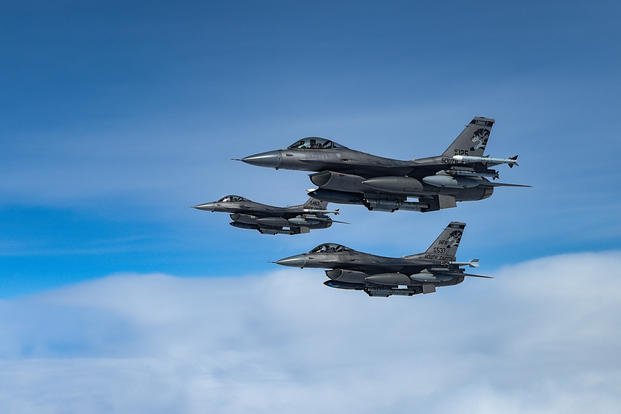The image depicts three sleek fighter jets, all oriented to the left in a precise formation. The lead jet is positioned higher, with two accompanying jets flanking it symmetrically lower and to its left and right. Each aircraft exhibits a streamlined, aerodynamic design in a gray-silver hue, featuring pointed noses and transparent glass cockpits perched on top. The jets are equipped with pronounced tail fins and smaller stabilizing wings, along with visible armament mounted on their sides and undercarriages. They soar high above the clouds, against the backdrop of a clear, vibrant blue sky with minimal cloud cover. The image's quality, with its sharp details and bright colors, suggests it could either be a highly realistic drawing, a sophisticated 3D rendering, or an exceptionally clear photograph, capturing the essence of modern aerial strength and precision.